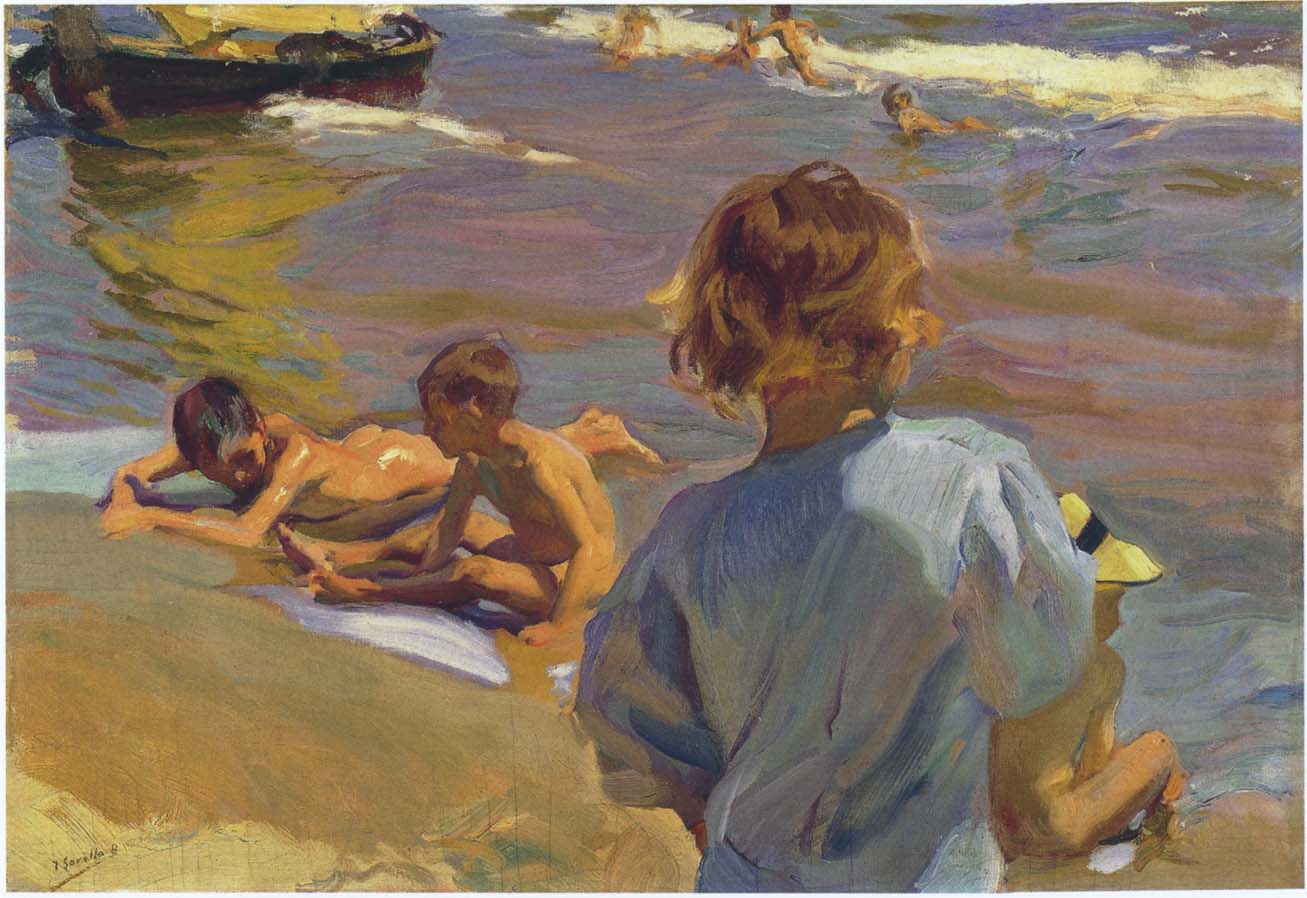This hyper-realistic painting captures a serene beach scene teeming with detail and life. Dominating the foreground, a child with long, blond hair, dressed in a blue shirt, stands with their back to us, surveying the animated shoreline. The beach is populated with several children, some in the water and others lounging on the sand. Prominently, there's a child in a sun hat sitting further to the right, and two more children closer to the center—one lying on his belly, and another seated upright. The water, an intricate mix of blue and grey hues, hosts four boys at play, their bodies glistening in the light that the painter skillfully captures. Gentle waves lap at the shore, creating a sense of motion. In the upper left corner, a wooden boat, indicative of maritime simplicity, rests in the water, manned by an adult figure. The scene is brought together with sophisticated textures and brushstrokes, imparting a bright yet calming atmosphere to the entire composition.